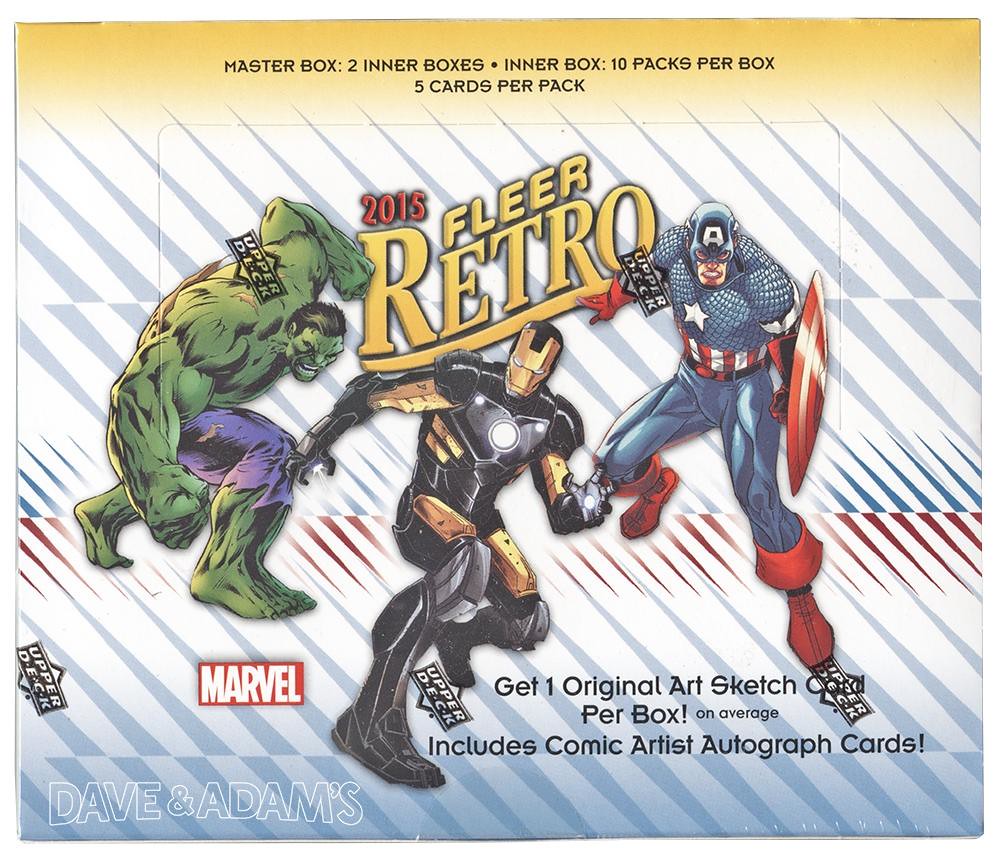This is a detailed advertisement-class image of a 2015 Fleer Retro box of Marvel action hero trading cards. The top text reads "Master Box, Two Inner Boxes, Inner Box: 10 Packs per Box, 5 Cards per Pack." The focal point of the design features three prominent characters: Captain America in his iconic red and blue suit, a black and gold variant of Iron Man, and the Hulk in green with purple shorts. The background is primarily blue with yellow trim and showcases the Marvel logo. The box also features an intricate design incorporating gray, blue, and red spikes on a white backdrop. The bottom text highlights "Get One Original Art Sketch per Box, Includes Comic Artist Autographed Cards." Additionally, there is a watermark on the bottom left, indicating Dave and Adams.